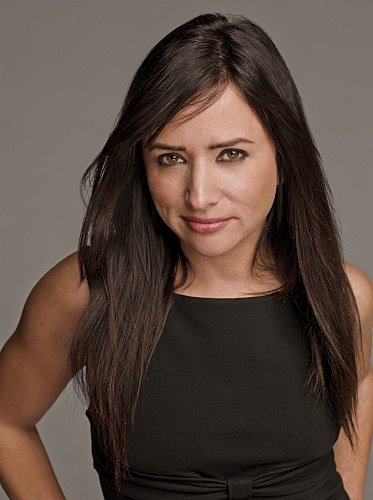This detailed photo captures Pamela Adlon in what appears to be a headshot-style publicity shot. She poses against a blank, grayish background, creating a minimalist backdrop that draws attention to her striking features. Pamela has long, straight dark brown hair that flows down to her chest, with bangs that frame her face. Her hair almost appears black, contrasting subtly with her complexion. Her light yet tanned skin highlights her facial features, including full lips, a larger nose, and expressive, wide-open light brown eyes accentuated with eye shadow and eyeliner. Looking straight into the camera with her chin slightly down and a subtle smirk on her face, Pamela's right side is a bit more forward, suggesting she's interacting with someone beyond the frame. She is dressed in a brown, sleeveless dress or top that ties around the center with a belt made of the same material, adding a cohesive touch to her look. Her shoulders are bare, and the detailed stitching of the dress's loop is visible, enhancing the garment's design.